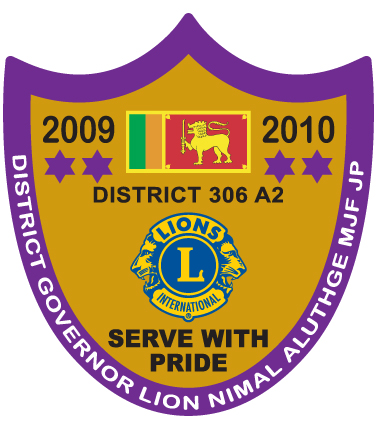The image depicts a crest-shaped badge with a purple border and a gold interior. At the top, it features the years "2009" on the left and "2010" on the right, each accompanied by two purple six-pointed stars underneath. In the center, there is a rectangular flag with red, green, and gold stripes, showcasing a lion holding a sword. Below the flag, the text "District 306A2" is displayed prominently. Underneath this, there is the Lions International logo, featuring two lion heads and a large "L" in the center. The badge also includes the slogan "Serve with Pride" in bold, black, uppercase letters at the lower section. Encircling the bottom curve of the purple trim is white text that reads "District Governor Lion Nemo Aluthghe MJFJP." The detailed imagery and text collectively highlight the badge's association with the Lions International Organization and its commitment to pride and service.